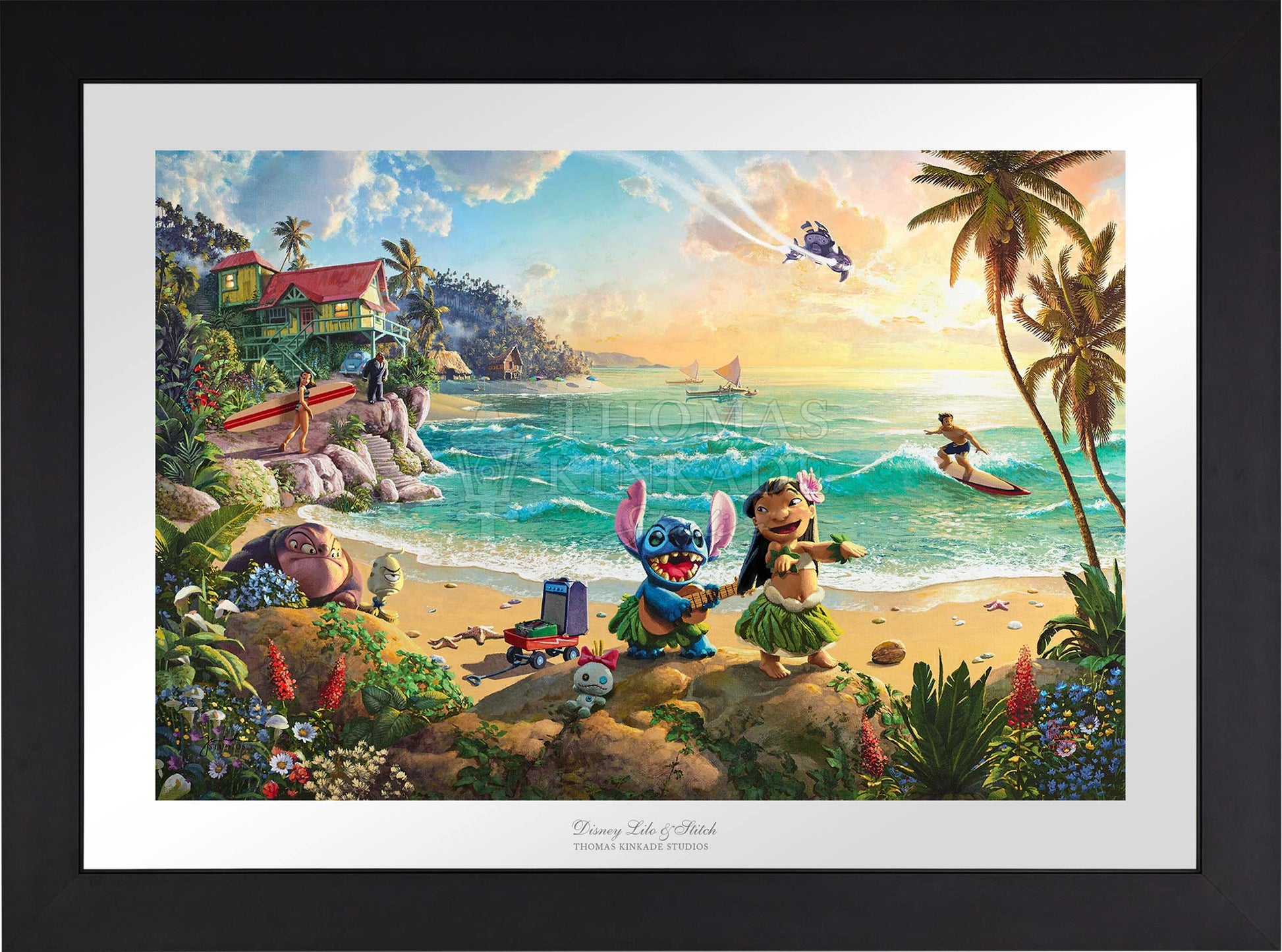This framed, vibrant lithograph by Thomas Kinkade Studios titled "Disney Lilo and Stitch" captures an enchanting Hawaiian beach scene. In the foreground, Stitch, the blue alien character, plays a ukulele while Lilo, the light brown-skinned hula dancer, dances beside him. Lilo sports a green hula skirt and pink flower in her hair. The corners of the illustration are adorned with lush island flowers and foliage. To the right, a graceful palm tree stands tall beside a surfer riding the waves. Nearby, a menacing man with a hunchback and a prominent chin lurks on the lower-left, casting a watchful eye. The background reveals rocks leading to a stilted beach house surrounded by palms, with another character, a girl carrying a surfboard, approaching. The vivid scene also includes other familiar characters from the movie subtly integrated into the background. The sky, filled with fluffy clouds and tinged with golden light, adds to the picturesque setting. At the bottom of the artwork, the titles "Disney Lilo and Stitch" and "Thomas Kinkade Studios" are elegantly inscribed on a white border, further emphasized by a surrounding black frame. The entire composition radiates a sense of whimsy and vibrant color, staying true to the joyous spirit of the beloved animated film.